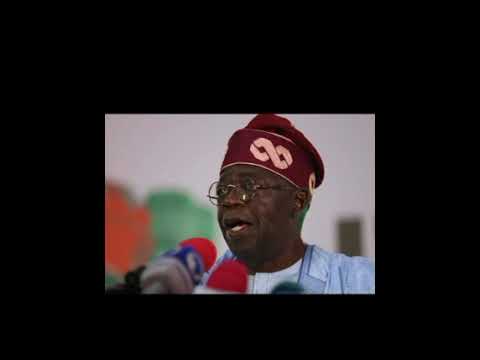In the center of a black horizontal rectangle lies a smaller, low-quality image of an African American man. The man's photograph, positioned just below center, shows him from the neck up, facing slightly to the right. He sports glasses and a traditional dark red cap adorned with a yellow symbol, possibly an infinity sign, around the band on his forehead. Dressed in a blue shirt or jacket over a white t-shirt, he appears to be speaking into two red microphones, suggesting he is at a press conference or giving a speech. The background behind him is blurred, adding focus to his figure. The black background frames the entire image on all sides, indicating the photo might be a video still or a compressed digital image.